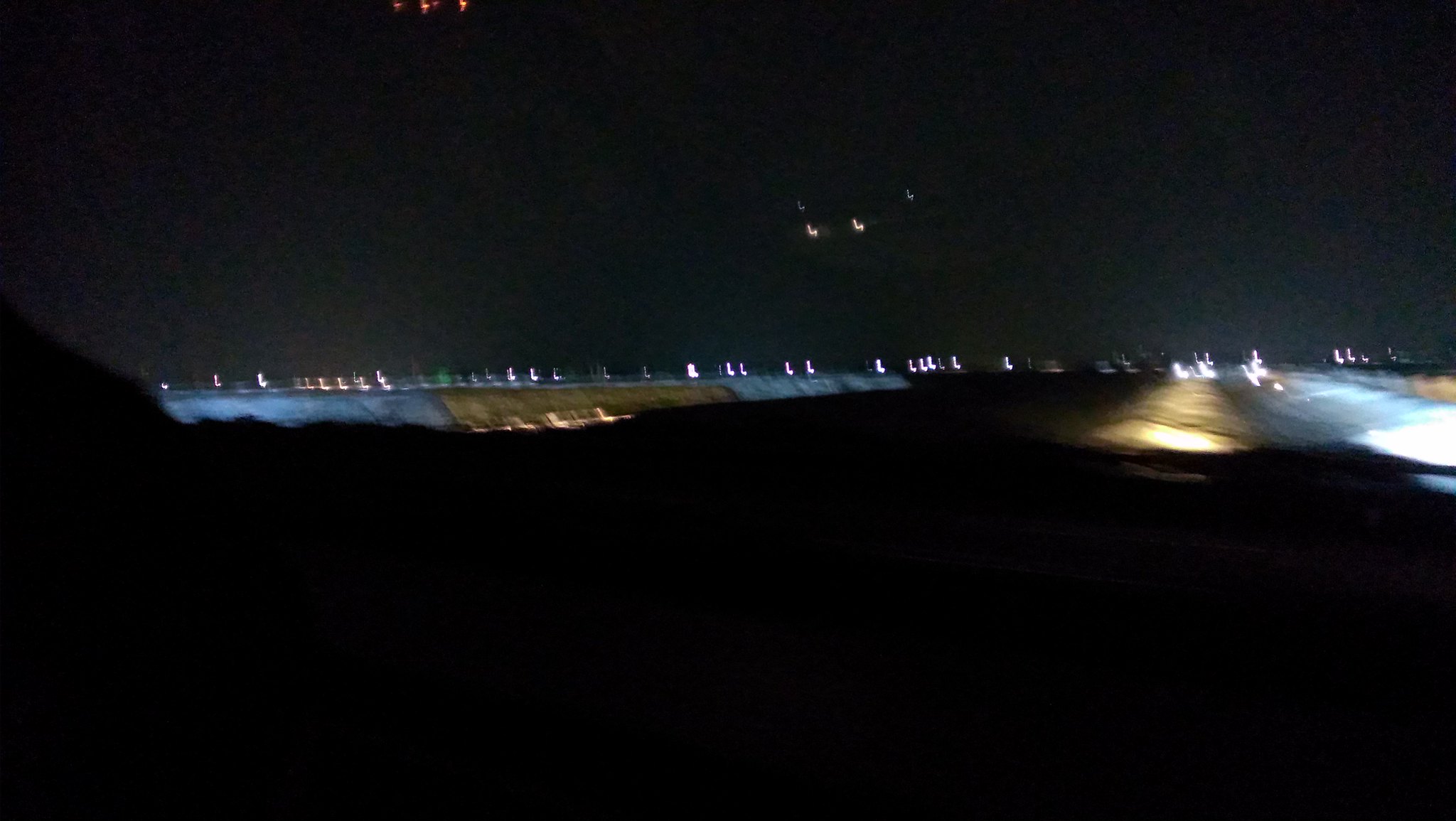In the foreground of this dark, night-time image, two-thirds of the space is consumed by a pitch-black expanse. Extending slightly to the right, a narrow strip of black land leads into the distance, creating a seemingly endless pathway. The upper right portion of the image features a brightly lit strip of land that appears to dip slightly in the middle, resembling a runway. The lights on this strip are predominantly white on the right side and orange on the left, with numerous lights stretching into the distant black sky, indicating proximity to an airport. Dominating the sky in the upper third of the image, slightly blurred and out-of-focus, an airplane is visible, distinguished by its two brightly lit jets and a subtly illuminated cockpit. Despite the overall fuzziness of the photo, the illuminated runway and the approaching airplane suggest a scene of an evening landing.